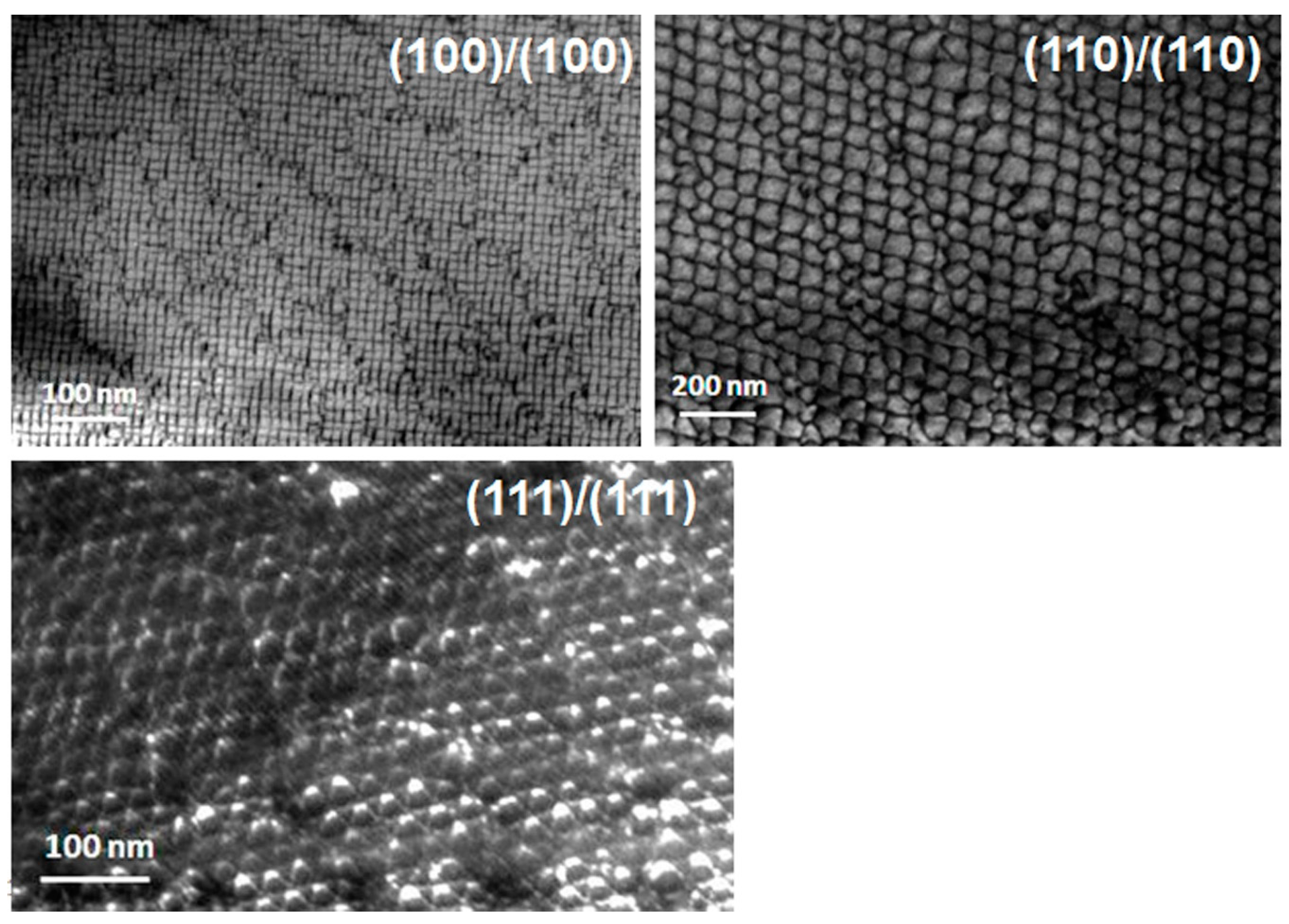The image comprises three black and white microscopic photos, each showcasing different scale-like patterns resembling snakeskin. The first image, located in the upper left corner, displays a series of very small square boxes pieced together to form a complete picture. It has a label "100 nm" at the bottom. The second image, positioned to the right, offers a close-up view with the label "200 nm." The third image, at the bottom, features thicker, more pronounced, bubble-like scales, labeled "100 nm." Each image appears uniform in grayscale, underlined, and contains a notation "100/100," "110/110," and "111/111" respectively, emphasizing different levels of magnification, specified by the nanometer (nm) measurements.